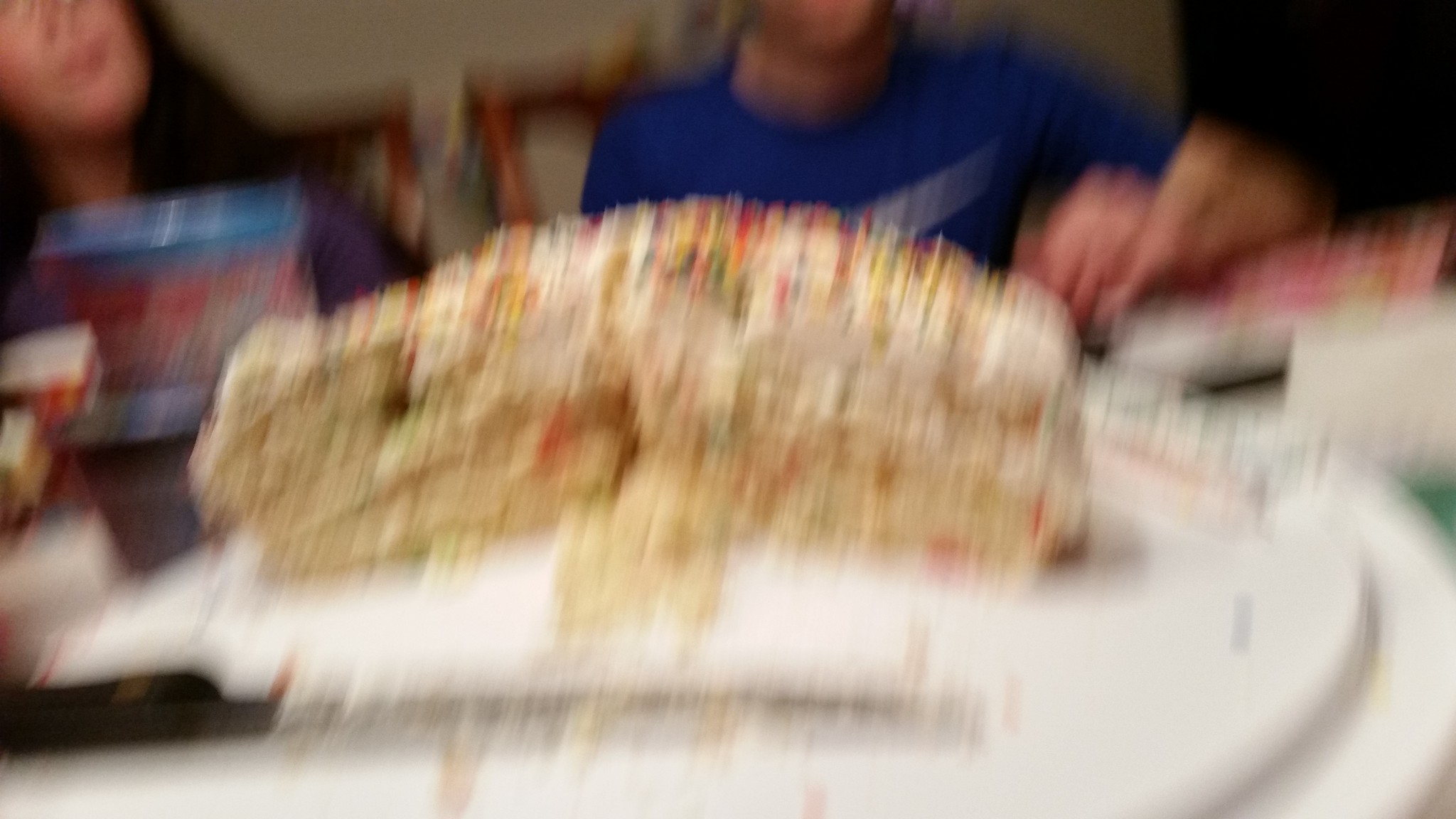This is a blurry photograph capturing what looks like a birthday party scene. In the image's foreground, a homemade vanilla cake with white icing and colorful sprinkles sits on a white plate. The cake, with over half of it already served, reveals a yellow interior. A black-handled knife with a silver blade is placed on the tray beside the cake, lying towards the right side. There are also two large, white plates holding additional pieces of cake.

In the background, two people are seated at a kitchen table. The person on the left, who has dark brown or black hair and wearing a purple top, appears to be a girl. She is possibly holding something in her hands. To her right sits a boy in a blue shirt featuring a white symbol on the front. Both are seated on partially visible brown wooden chairs. The wall behind them is a light gray color, and the top of their heads is cropped out of the image. The scene, indicative of a gathering or celebration, is set in a kitchen with various items scattered on the table and a darker section towards the upper right corner.